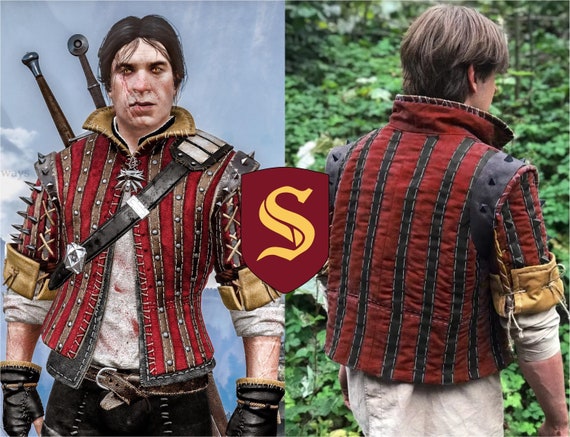The square image is a split-screen composition, blending photographic realism with artistic illustration. At the center, a burgundy shield featuring a prominent golden S acts as the focal point. On the left side of the image, there is a detailed illustration of a dark-haired, 3D-rendered warrior. This character, depicted in front view, dons a medieval-inspired outfit that includes a red and brown vertically-striped jacket with black spikes on the shoulders, a white long-sleeved shirt, black gloves, and black pants. His weathered appearance is accentuated by black hair parted in the middle and two swords strapped to his back, one on each shoulder, adding to his battle-worn look. On the right side, there is a corresponding real-life photograph of the back of a Caucasian male, who wears a similar red and black decorative vest. He stands against a backdrop of lush green vegetation, further drawing a parallel between the animated character and its real-world counterpart. This juxtaposition highlights the artistic translation of the medieval attire from fantasy to reality.